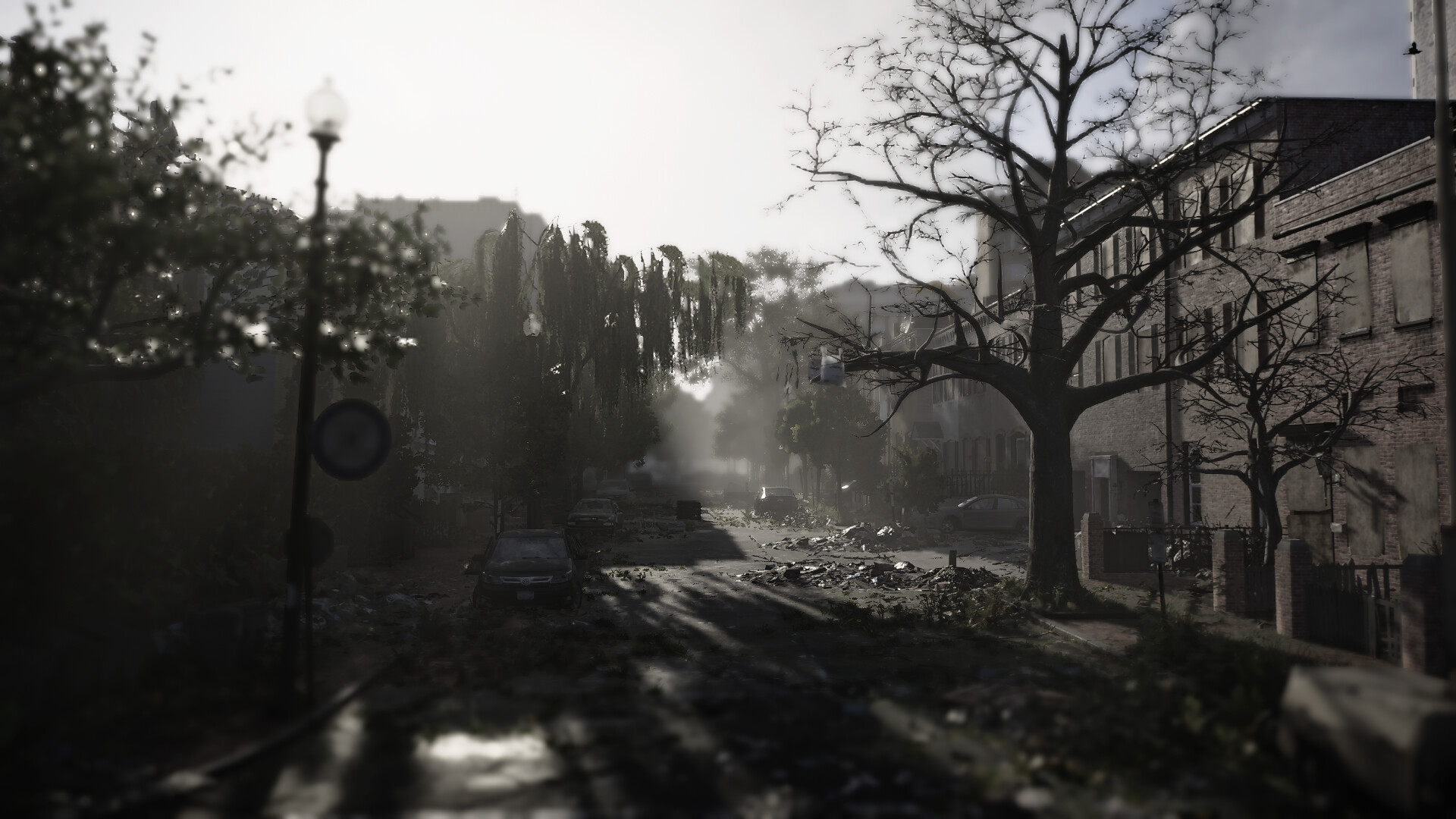The image depicts an abandoned city street rendered in a computer-generated, dystopian style, with the predominant aesthetic being black and white. The scene features a row of brick buildings on both sides of the street, emphasizing a sense of desolation. The ground is littered with garbage and debris, and the asphalt appears broken and deteriorated. Several cars are parked along the street, characterized by their dusty windows, indicating a prolonged lack of use.

On the right side of the image, there is a dead tree, starkly contrasting with the two trees on the left, which still have some leaves, offering a slight hint of vibrancy against the grey backdrop. The leaves of those trees might possess a very pale green hue, though the overall palette remains muted. A streetlamp extends skyward, its light conspicuously off, adding to the abandoned atmosphere. There is also a circular plaque hanging nearby, likely meant to provide some sort of information.

Brilliant sunlight pierces through the scene, creating dramatic shadows across the buildings, trees, and other objects, adding to the eerie, deserted ambiance. Despite a faint hint of a bluish sky at the top, the overall impression remains one of stark abandonment and artificiality, characteristic of a meticulously designed computer-generated image.